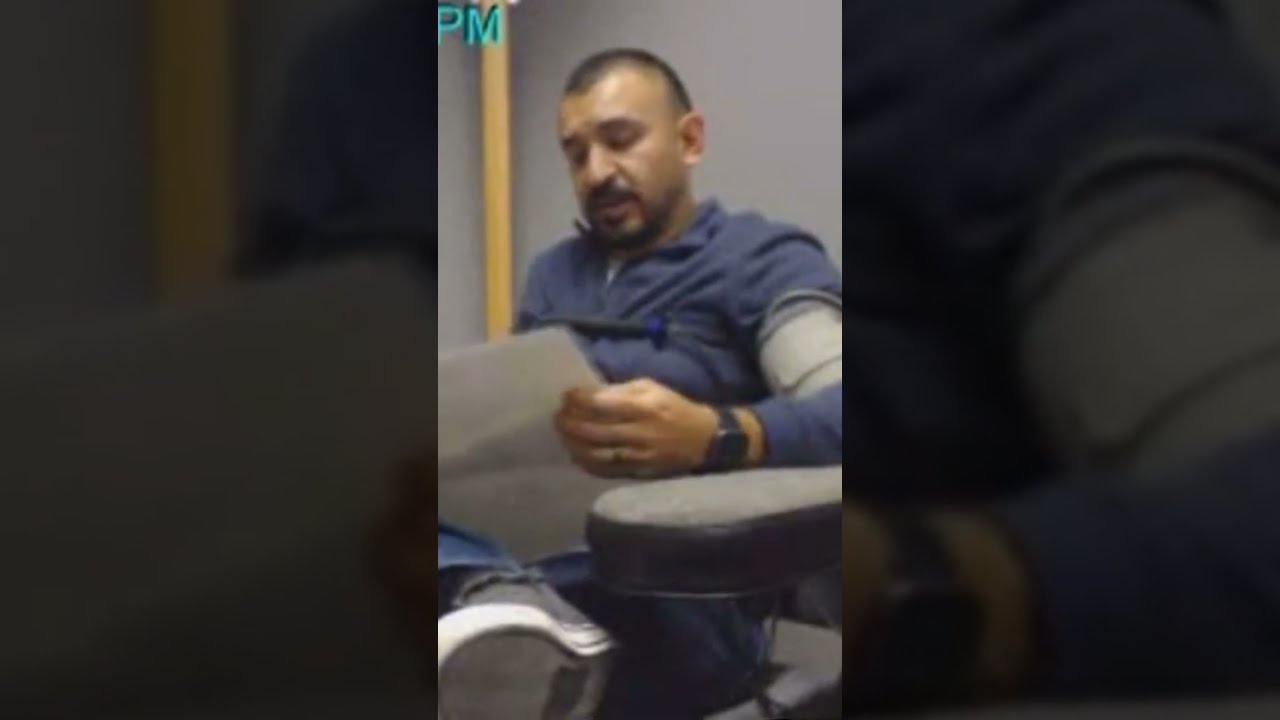The photograph captures a detailed and somewhat somber scene of a Hispanic male, approximately 40 years old, who is seated with his left leg crossed over his right. The focal point is the man, who is gazing down intently at a piece of paper he holds in his left hand. He is dressed in a blue sweatshirt with long sleeves, beneath which a blue cast or pressure sleeve is visible on his left arm, suggesting a medical procedure or health check. His outfit is completed with blue jeans and gray sneakers with white soles. 

The man has a beard and mustache and wears a black watch and wedding band on his left wrist. The background features a gray wall accented with a light wood-colored corner and a yellow line on the left side. In the top left corner, the letters "P.M." are prominently displayed in blue, hinting at either the time of day or a timestamp. The close-up blurs to the left and right of the image emphasize the man's engrossed posture as he reads the paper, adding to the scene's intimate and contemplative atmosphere.